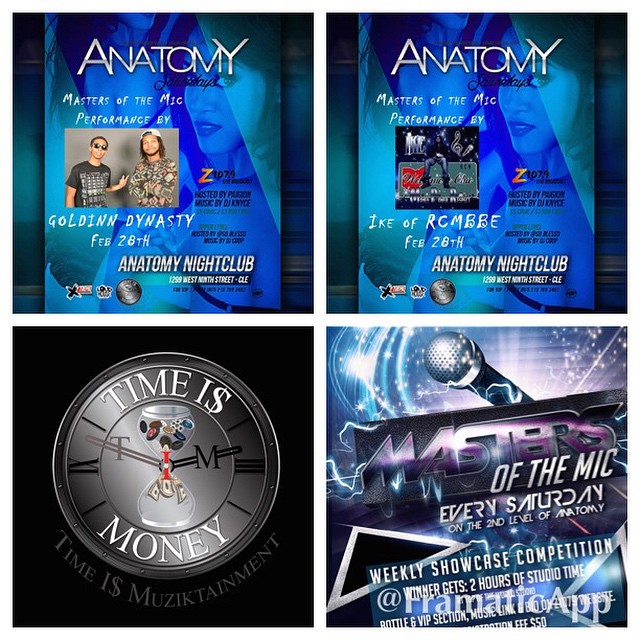This image features a grid of four promotional flyers for events at Anatomy Nightclub, forming a square with two flyers on top and two on the bottom. The top two flyers share a blue theme with silver lettering, both titled "Anatomy Saturdays." These posters are advertising different events, highlighting DJs and performances with a background image of a woman. In the bottom left corner, there is a flyer with a green clock featuring an hourglass at its center, emblazoned with the phrase "Time is Money" and "Time is Music" against a black background. The bottom right corner displays another flyer, "Masters of the Mic," advertising a recurring event every Saturday on the second level of Anatomy Nightclub, with a background of a microphone and sparkles.